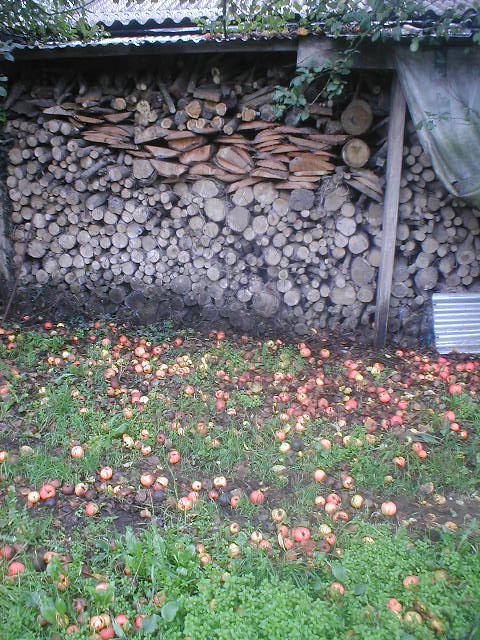This photograph captures a well-stacked woodpile under a weathered lean-to shed with a corrugated metal roof. The shed, supported by timber posts, is fully loaded with various sizes of chopped wood, from smaller tree rounds at the bottom to rectangular slabs at the top. The wood appears to range in age and dryness, with older, darker pieces at the bottom, dry gray ones in the middle, and newer, fresher logs on top.

In the foreground, a lush but patchy grassy area is littered with numerous apples, varying in ripeness and color from red to yellow. Some apples appear to be rotting, hinting at the proximity of an apple tree. Additionally, green leaves and branches from nearby trees hang over the shed, adding a touch of nature to the scene.

A closer inspection of the right side reveals a brown timber pole supporting the metal roof, along with a worn, grayish canvas that seems to be tied to the structure. The overall ambiance of the image suggests a preparation for winter, with the woodpile ready for use in a fireplace or potbelly stove.